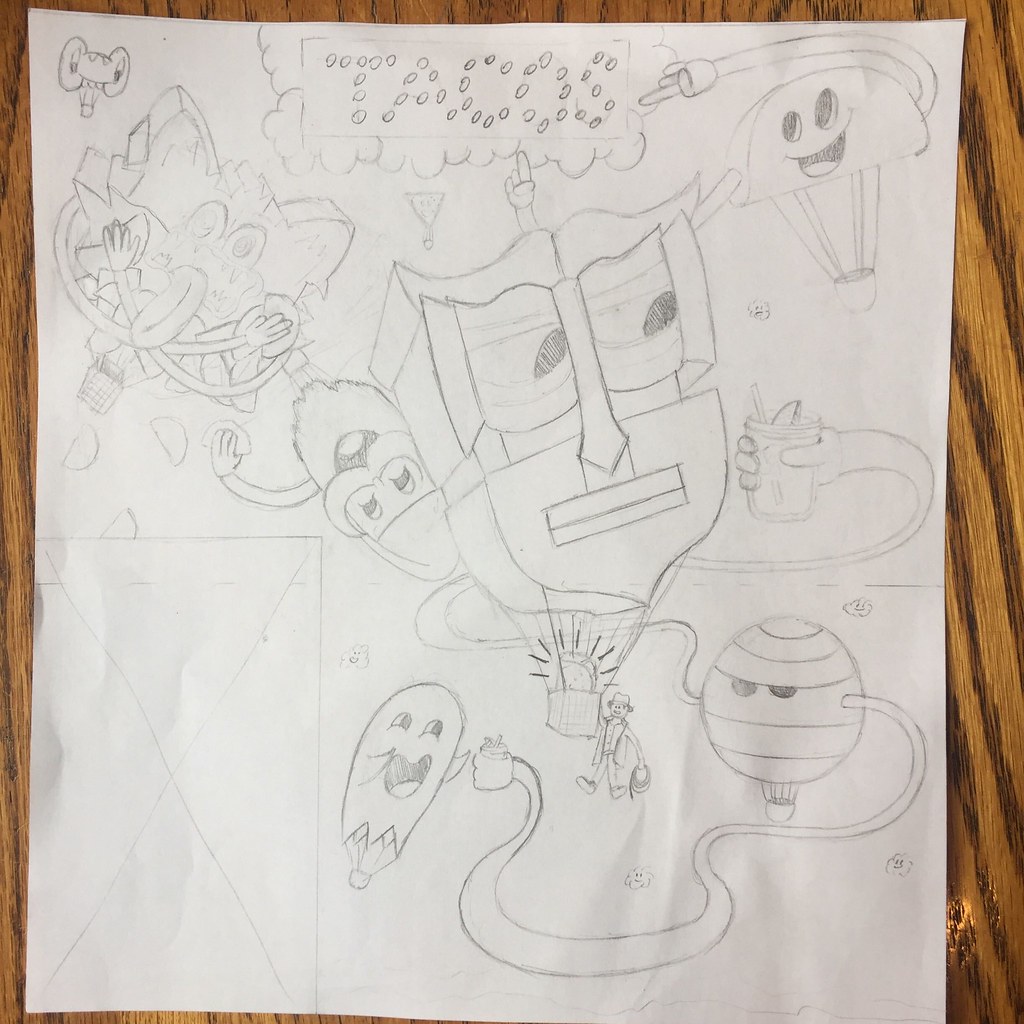This photograph showcases a slightly crumpled piece of paper resting on a light brown wooden surface, adorned with prominent, darker brown vertical wood grain stripes. The paper features various pencil sketches depicting whimsical, cartoonish characters, each with distinct faces and appendages. Central to the artwork is a detailed rectangle at the top, bordered by cloud-like figures, containing circles that spell out the word "TACOS." Among the illustrated characters, one appears shaped like a taco shell, while another holds a drink. These imaginative beings resemble hot air balloons, complete with baskets hanging beneath them by strings. In the lower left-hand corner of the paper, a notable rectangle bears an 'X', adding an enigmatic touch to the overall playful and creative scene.